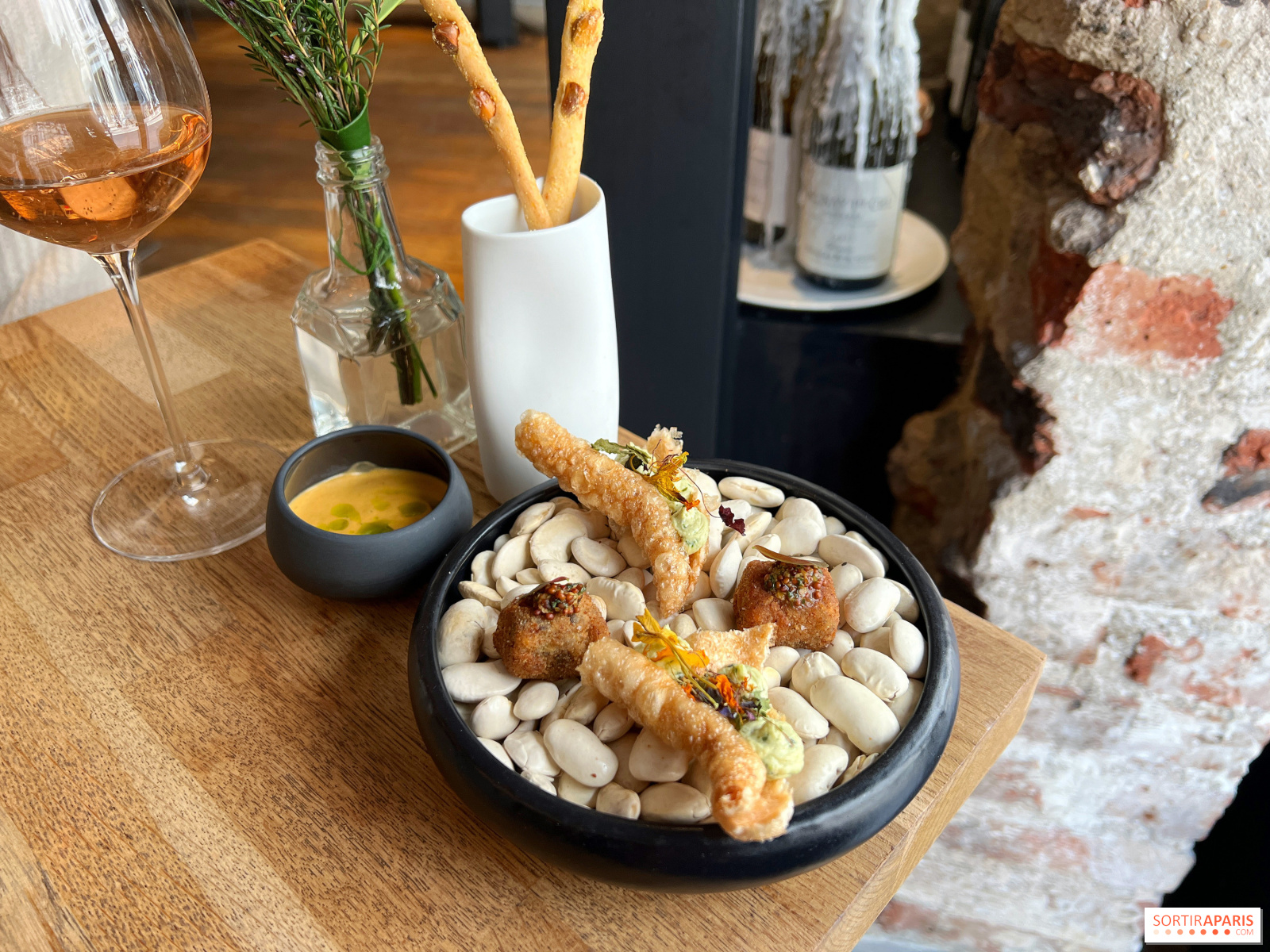The photograph captures a meticulously arranged meal on a light wooden table. At the center of the small wooden table sits a dark blue dish containing a bean dish, topped with a fried element and accompanied by two brown and beige croquettes. The plate is adorned with bright yellow, orange, purple, and green flower garnishes. This dish is presented atop decorative rocks. Beside it is a smaller dark blue dish filled with a vibrant yellow liquid, likely a sauce or soup. 

To the left, a clear wine glass holds a light pink liquid, suggestively a rosé wine. The table also features a white vase containing two breadsticks, and a clear vase filled with water and topped with a green plant, its upper part extending out of the frame. In the background, the scene is complemented by two wax-covered wine bottles against a column of brick, adding a rustic touch to the elegant setting.